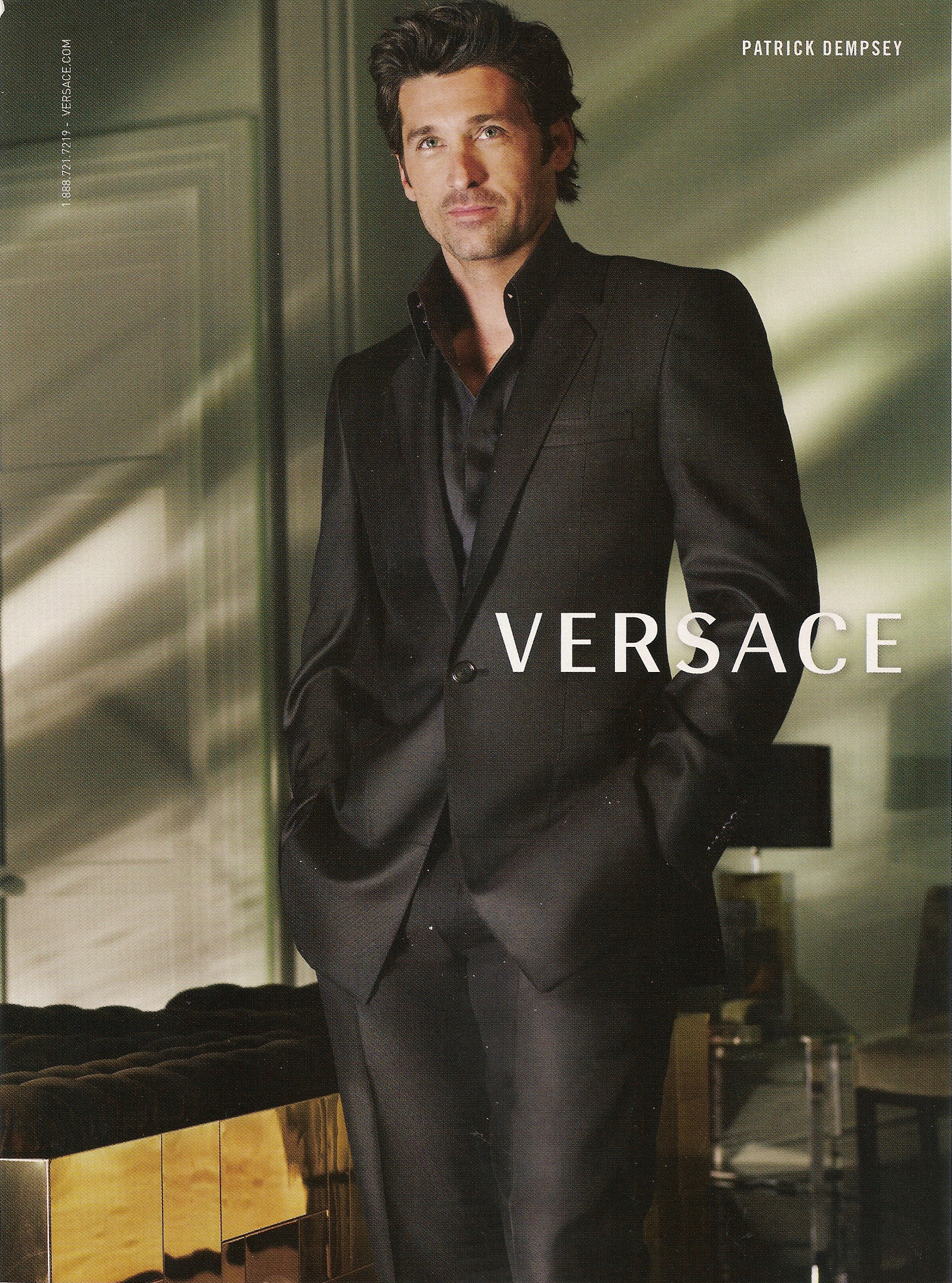Actor Patrick Dempsey stands confidently in this sophisticated indoor setting, featured in a stylish Versace advertisement. Dempsey, known for his dark, professionally combed hair and distinct low-profile goatee, exudes elegance in a finely tailored, black suit paired with a black collared shirt. His hands rest casually in his pockets as he gazes directly ahead. The room, illuminated subtly from the side, casts dramatic shadows across its white walls, creating a moodish atmosphere. 

Key elements behind him include a mix of mid-century modern furniture: a black-shadowed door, a light brown and cream-colored sofa, a table with a lit lamp featuring a black shade and metallic base, and a minimalist bench with a light brown structure supporting a black cushion. The arrangement of these pieces adds to the chic yet understated environment. Versace's name, in white sans serif font, is prominently displayed to the right of Dempsey, emphasizing the luxury brand's association with high fashion. At the top right of the image, “PATRICK DEMPSEY” appears in all capital letters, reinforcing his identity and star power in this vertical composition that could serve as a magazine spread or an eye-catching billboard.